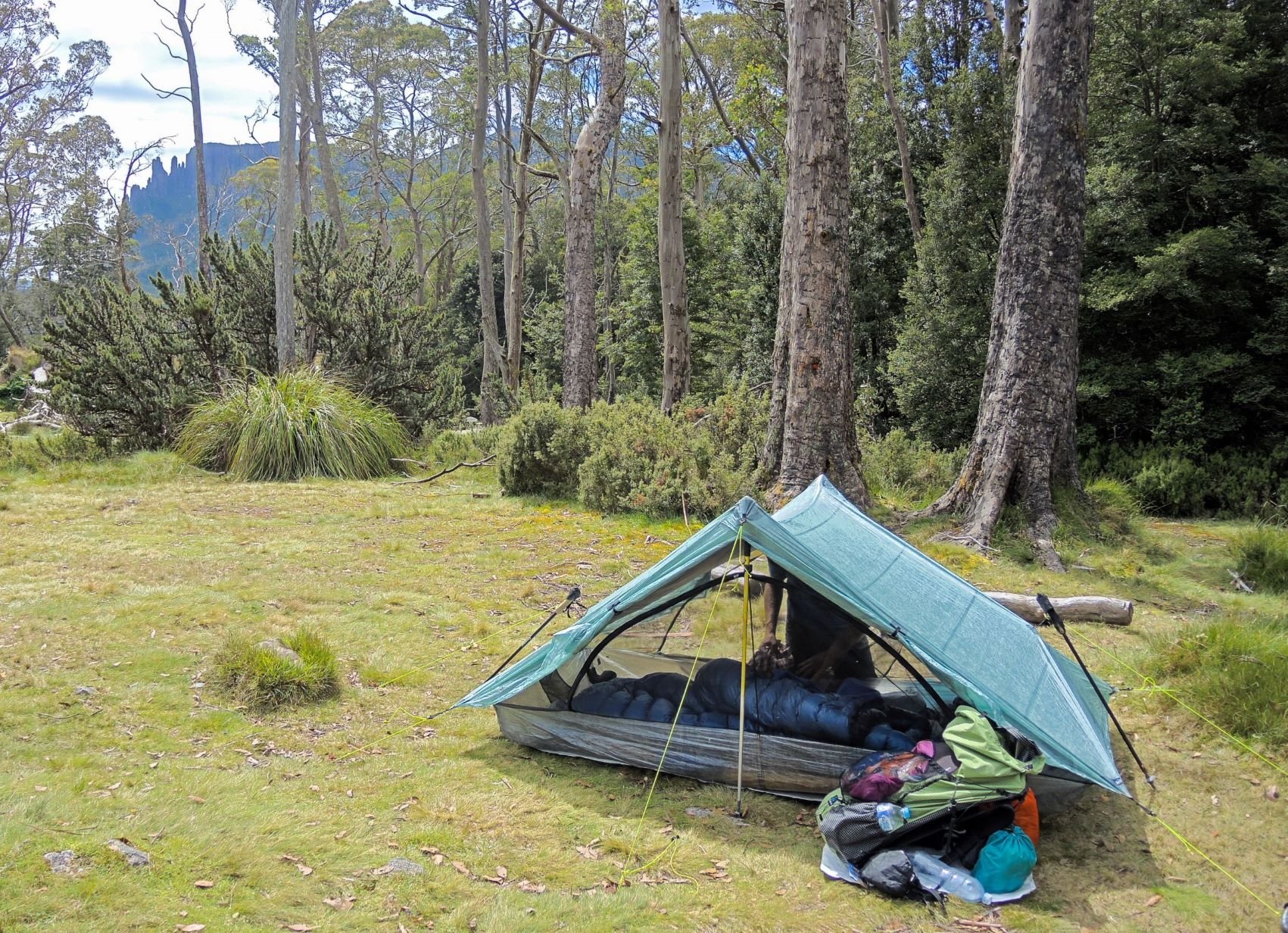The photograph captures a vibrant outdoor campsite scene during the daytime. Set in a grassy area bordered by a dense wall of vegetation, including towering brown tree trunks and green pine trees, the focal point is a tent located near the bottom right corner of the image. The tent features a prominent A-shaped roof in a light blue-green color and appears sturdy with bungee cords anchoring it to the ground. In front of the tent lies a neatly stacked assortment of camping equipment, including a colorful pack with hints of pink, green, blue, and orange, as well as a couple of water bottles. Notably, there’s a dark blue sleeping bag inside the tent, which is slightly transparent at the bottom and reveals a man of African descent adjusting the bag. The top portion of the image presents a clear blue sky dotted with thick clouds and a view of distant mountains in the upper left corner, adding a serene and majestic backdrop to the camping setting.